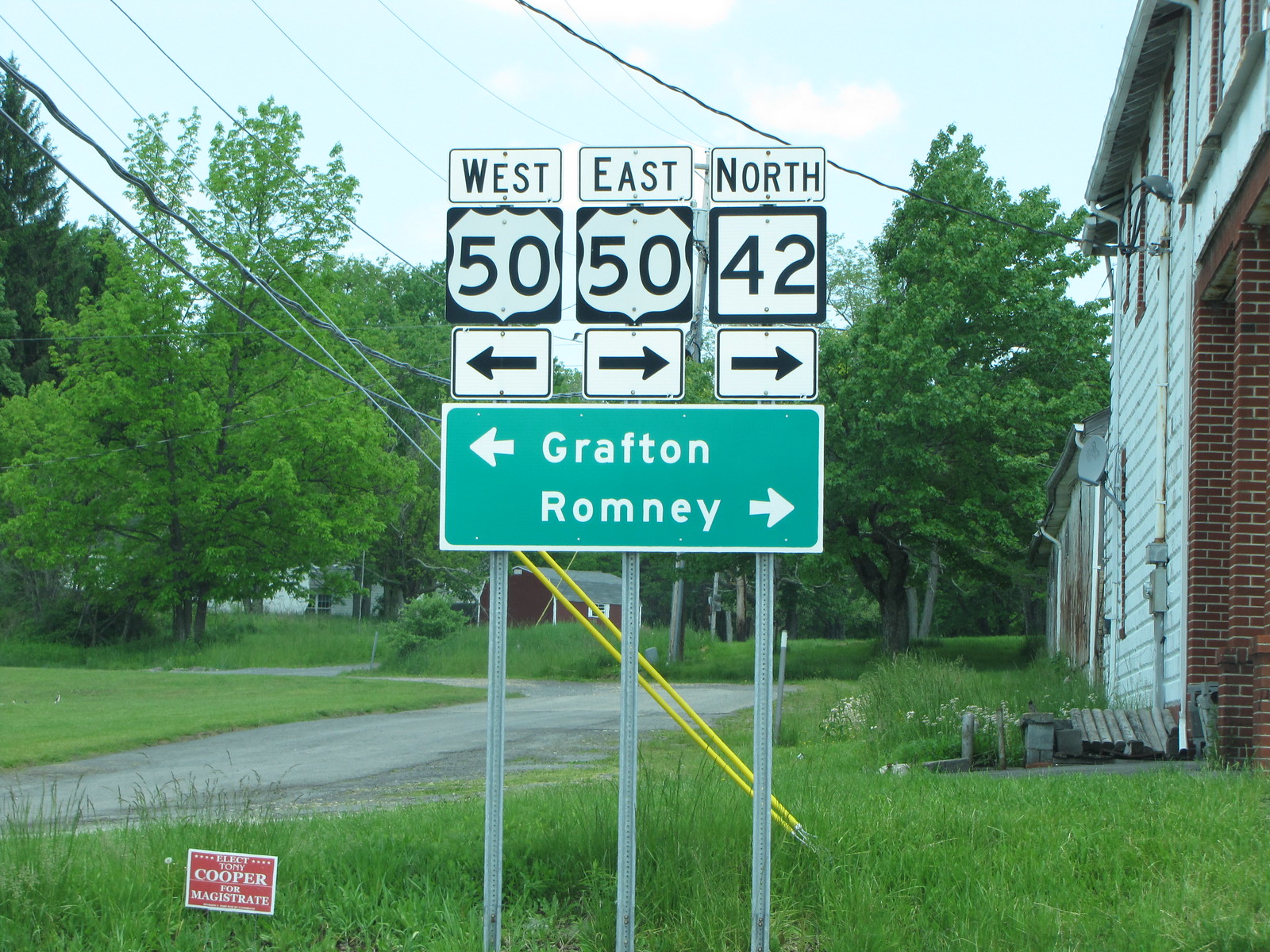A quaint roadway stretches ahead with tall grass lining its edges, partially obscuring a small red sign that appears to read "Cooper." Long yellow lines ascend from the ground to the power lines above, while a black cable snakes toward a small brick building with white wooden trim, showcasing some exposed electrical components. Prominently displayed at the roadside, three tall posts support a series of directional signs. The bottom sign is green with black and white borders, featuring white letters that indicate "Grafton" with a left-pointing arrow and "Romney" with a right-pointing arrow. Additionally, the sign directs travelers with "West 50" pointing to the left, "East 50" pointing to the right, and "North 42" also pointing to the right.